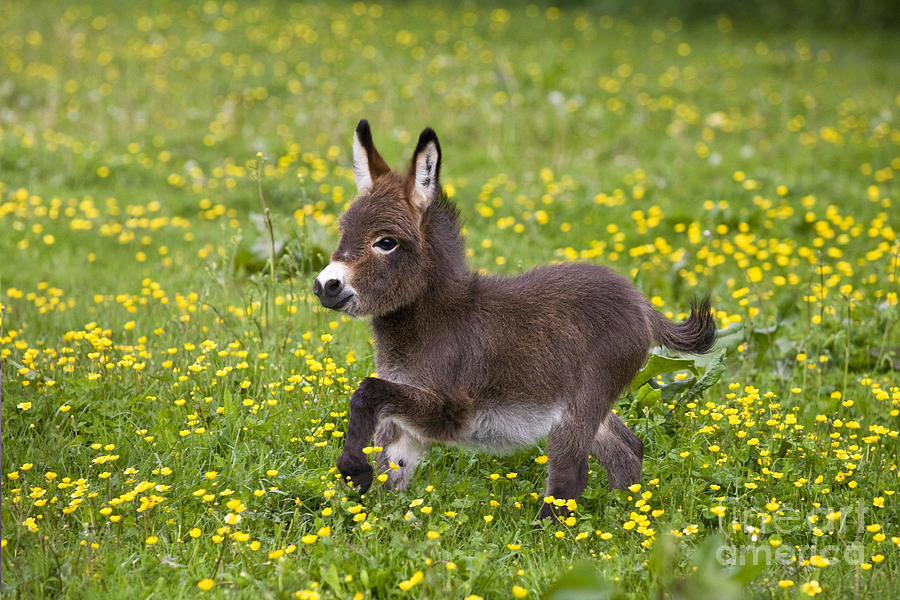In the midst of a lush field with rich green grass dotted with vibrant yellow flowers, a miniature baby donkey captures the scene's essence. This diminutive creature, looking so small it could be mistaken for a creation of artificial intelligence, stands out with its striking details. The donkey's coat is a mix of grayish-brown, with a fuzzy texture, and white patches. Its ears, brown on the outside and white on the inside, stand alert and upright, giving an impression of keen curiosity. 

The donkey’s black eyes, accentuated by white markings, bring a calm and placid expression to its face. Its muzzle is predominantly white with gray markings around the edges, leading to a black nose with distinct nostrils. The contrast continues with a white furry belly and dark brown to black hooves. One front leg is raised and bent at an angle, suggesting movement, while the other legs support its body in a dynamic pose. 

Further enhancing its appeal, the short, bushy tail sticks straight out, partly white underneath, adding a playful touch to its appearance. In the background, the field continues to blur slightly, creating depth, while some green plant matter in the foreground also blurs, focusing attention on the beautifully detailed miniature donkey in the center of the image.